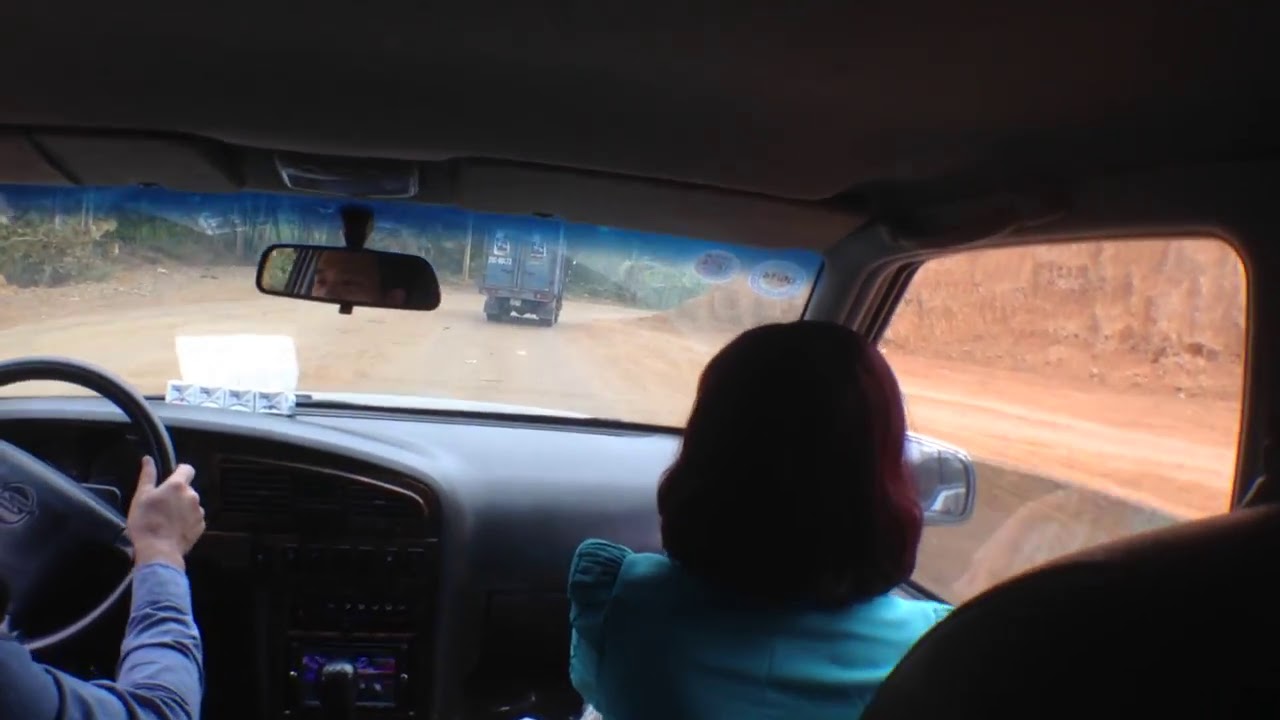This detailed caption consolidates the shared and repeated elements from all four descriptions:

The photograph, taken from the back seat of a car, captures a scene on a rugged, dirt road in a foreign country. The car is driven by a man with pale skin, visible in the rear-view mirror and identifiable by his blue long-sleeve shirt and hand on the steering wheel. In the passenger seat, a woman with short, red hair and wearing a blue or turquoise dress sits calmly. Outside the car, through the dusty windshield and passenger-side window, the landscape reveals a hilly area with numerous trees and a dirt pile in the distance. Directly in front of the car, a small green truck, possibly a box or garbage truck, equipped with mud flaps, travels along the road. Inside the car, a standard CD player and black steering wheel are noticeable. The overall scene is captured in broad daylight, with the rugged terrain and natural surroundings providing a vivid backdrop.